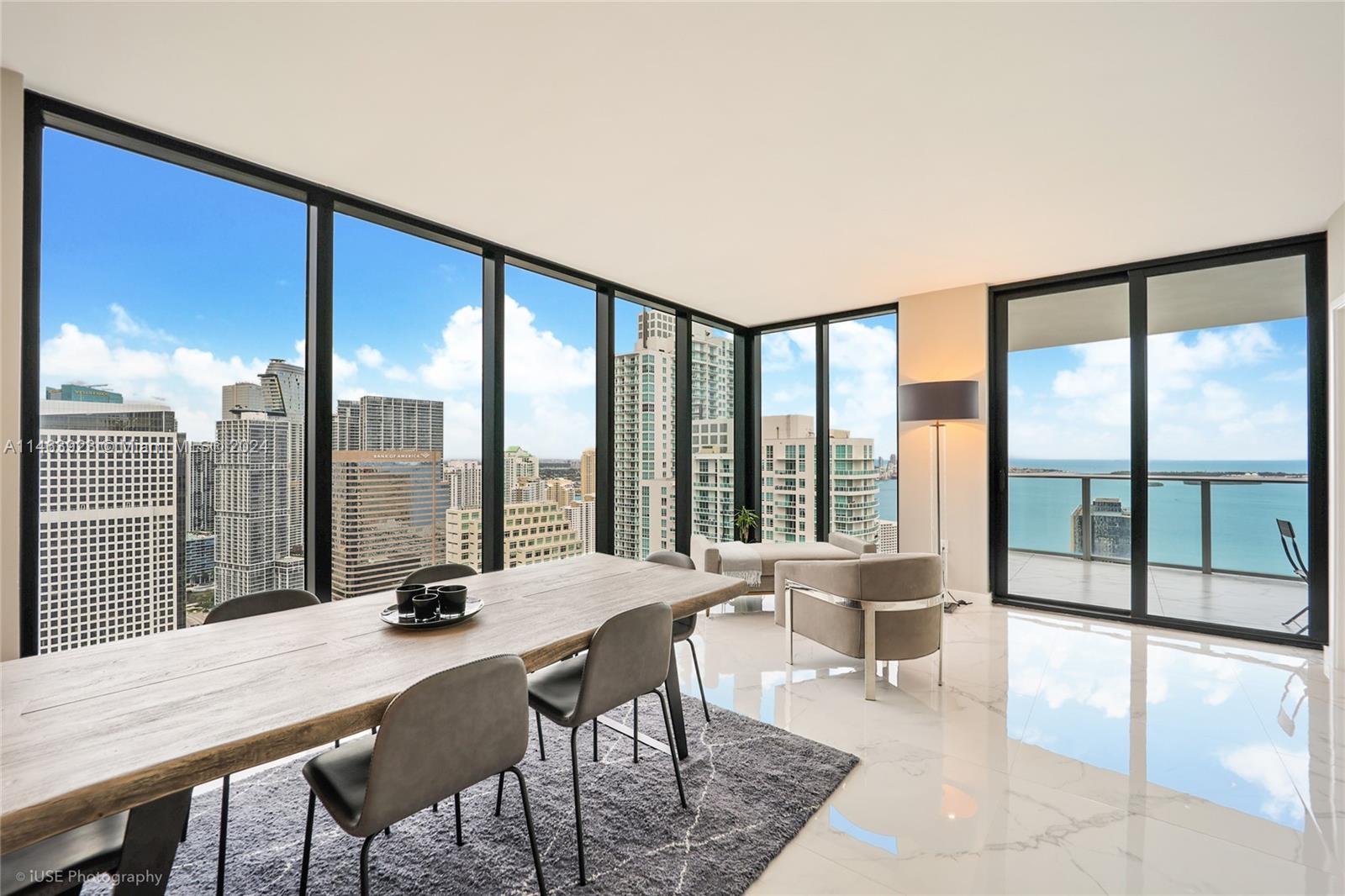The image depicts a meticulously designed modern interior space, possibly computer-generated, resembling a luxurious apartment or office located in a very tall building. The room is characterized by its expansive floor-to-ceiling glass windows framed in black, allowing ample natural light to flood in and providing stunning views. Outside, the daytime scenery features a blue sky scattered with white, fluffy clouds, the tops of nearby skyscrapers, and a body of water with a distinct blue-green hue. Inside, the decor exudes sophistication with white marble floors exhibiting fine veining, white walls, and a white ceiling. The centerpiece is a long, rectangular wooden dining table situated on a stylish grey area rug, surrounded by modern, armless grey chairs. The table is adorned with a serving platter and cups. Beside one of the large windows stands a lit floor lamp with a dark shade, illuminating a cozy seating arrangement including a rounded chair and an accompanying ottoman. Additionally, a desk with a modern chair is positioned in a corner, contributing to the functional yet elegant ambiance. The overall design style emphasizes sleek interior architecture, blending comfort with contemporary aesthetics.